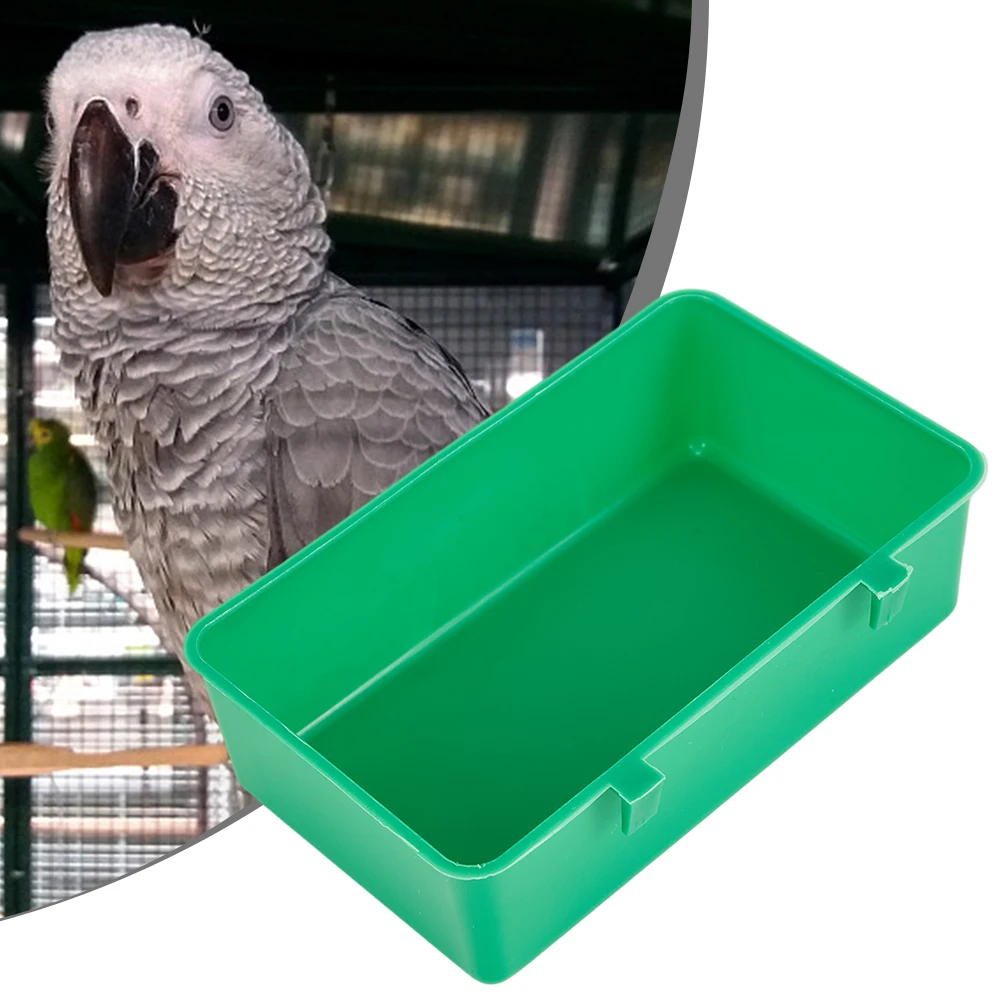This photograph features a detailed close-up of two birds inside a cage. The primary focus is on a large white-and-gray parrot perched on a small wooden stick. The parrot is distinguished by its gray body, white head, and prominent black beak. Positioned behind the parrot is another bird, characterized by its vibrant green body and a head that blends yellow and green hues, with a subtle gray beak. In the foreground, a dark green, rectangular plastic feeding dish, conspicuously empty, is attached to the cage via two hooks. The cage itself is gray, contrasting with the bright daylight visible through a potential skylight above. The background also reveals the second bird, slightly blurred and adding depth to the scene.